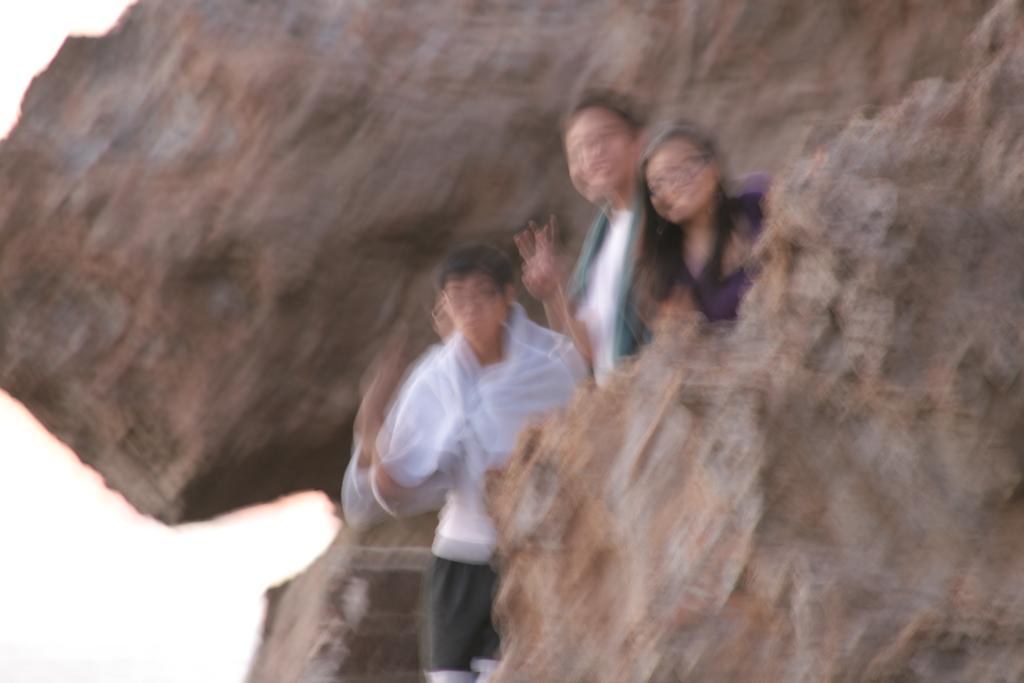A blurry photograph captures a scene in motion against the backdrop of a large, textured, brown boulder with various hues of brown, invoking a sense of ruggedness. Amidst the blurred setting stand three figures, slightly obscured but discernable. On the left, a young boy with black hair and glasses is dressed in a white shirt and black shorts. Central to the group, an older woman with black hair wears a white top underneath a green jacket. On the right, a young girl with black hair is clad in a black top. The overall motion blur lends a dynamic and somewhat abstract quality to the image, leaving the viewer to imagine the details amidst the evident action.